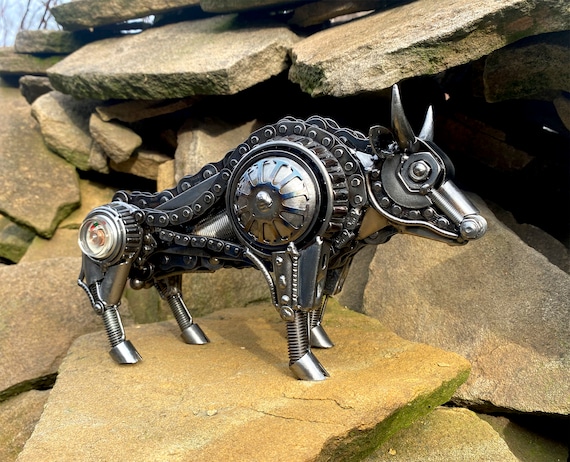In this outdoor photograph, a meticulously handmade steampunk-style bull sculpture takes center stage, crafted entirely from metallic bike chains, springs, and various other metal components. The bull, adorned with two curved horns and intricate detailing formed from rivets or screws, faces towards the right. It stands proudly on a light brown, flat stone. The scene is set against a backdrop of stacks of similar flat stones, covered in patches of green moss, creating a striking contrast with their gray and light brown hues. Bare tree branches stretch across the top left corner under a pale blue sky, framing the mechanical marvel with a natural touch.